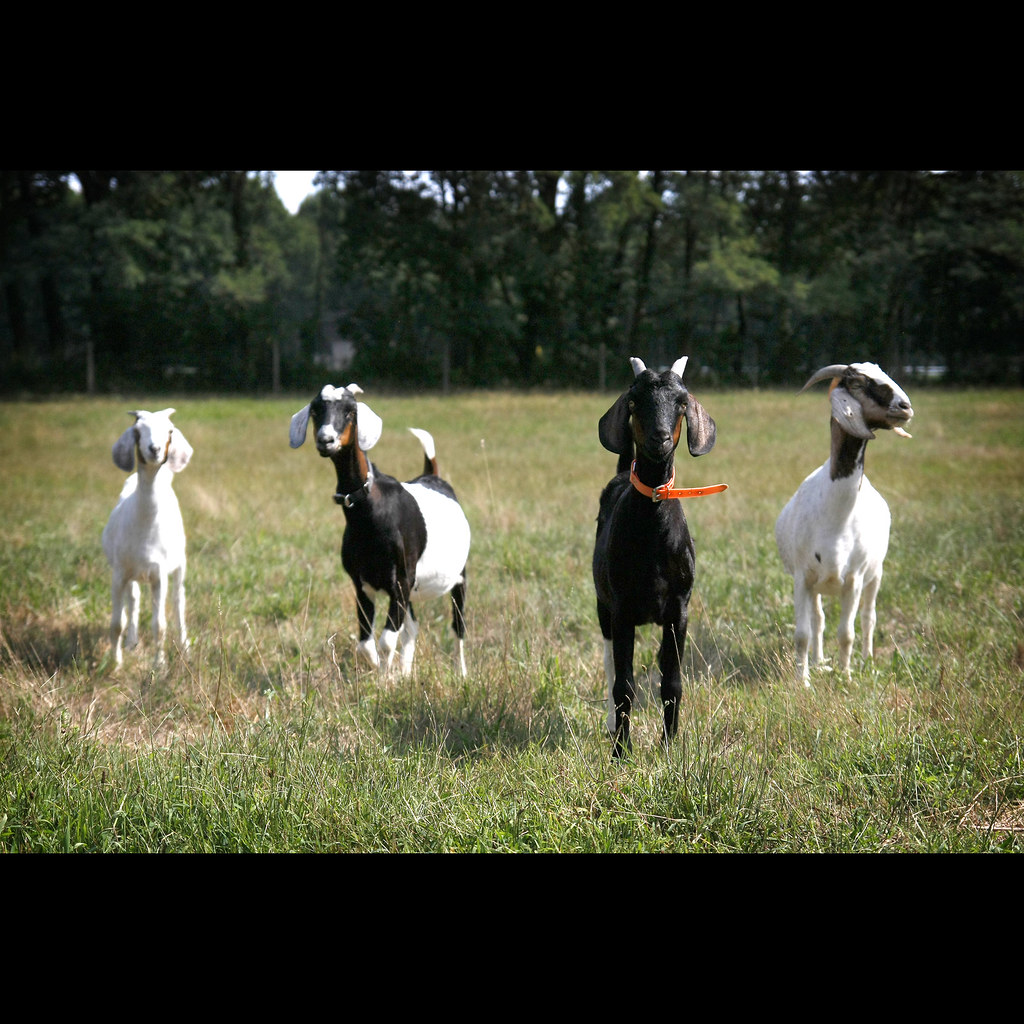The image depicts a flat, grassy field with four distinct goats as the main focus. In the background, there is a dense array of tall, dark green trees and other lush greenery, slightly blurred to accentuate the foreground. The goats are standing in a line, all facing and looking directly at the camera with their floppy ears and bulging, beady eyes.

On the far left is a mostly white goat. To its right is a uniquely colored goat with a white belly, a black and brown chest and neck, and white ears. Its nose and the area on top of its head are also white. Next in the line is a black goat wearing an orange collar, with stark white horns. Finally, on the far right, there is another goat which appears to be mostly white but features some black and gray markings on its face and neck. The contrast of their coats and the uniformity of their gaze create a striking visual against the serene green backdrop.